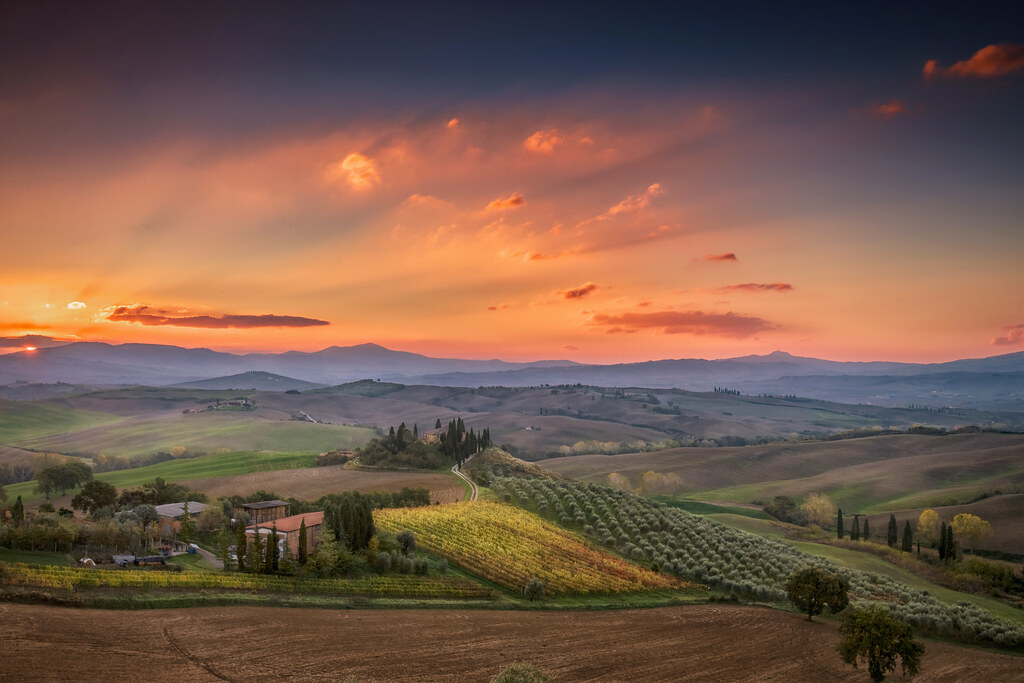This is a gorgeous, detailed digital painting of a tranquil farm landscape at sunset. The sky above is a blend of orange and dark gray hues with wispy clouds scattered throughout. In the distance, grayish mountains or rolling hills add depth to the scene, contrasting with the lush, green acres in the foreground that clearly depict well-manicured, plowed fields. Central to the painting is a patchwork of farmland, including fields that might be growing corn, lettuce, and other crops beneath the soil, all arranged neatly in rows. Scattered trees and shrubs provide additional texture and framing throughout the scene, with noticeable clusters in the lower right, middle, and left portions of the painting. The distant houses dotting the landscape add a touch of human presence to this serene, idyllic setting. Overall, the painting beautifully captures the peaceful and tranquil essence of nature, showcasing the extensive fields, rolling hills, and the grandeur of an open sky at dusk.